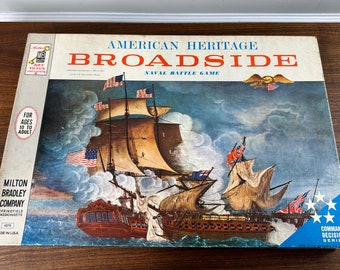This image features the American Heritage Broadside game, prominently displayed on a dark brown wooden table with a white wall in the background. The title "American Heritage" is printed in blue, and "Broadside" in red, both set against a white background. Below the title is a dramatic depiction of a naval battle between two large brown ships with light brown sails. One ship, flying American flags, engages another vessel adorned with a red and blue flag, suggesting a historical conflict like the War for Independence. The turbulent sea and stormy, cloud-filled sky add intensity to the scene. To the left, symbols and text indicate the game is suitable for ages 10 to adult, and it is produced by the Milton Bradley Company.